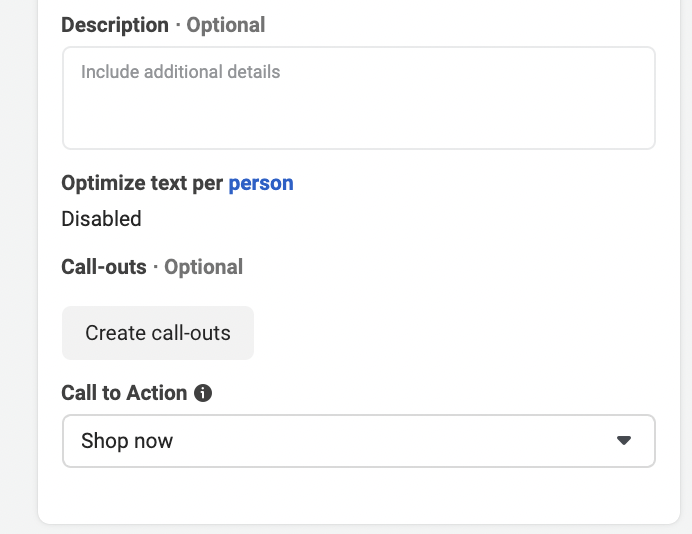A screenshot of a user interface with a predominantly white background bordered by light gray edges. At the top of the screen, the word "Description" is displayed in black, followed by a gray dot labeled "Optional." Below this is a text box with the placeholder text "Include additional details." Further down, the phrase "Optimize text per" appears in black, with the word "person" highlighted in blue, and the status "Disabled" indicated underneath. 

Next, the word "Callouts" is shown in black, accompanied by another gray dot labeled "Optional." Directly below is a gray button labeled "Create Callouts." The section titled "Call to Action" follows, featuring a clickable information icon beside it. Underneath this section is a drop-down menu labeled "Shop Now," which includes a downward-facing arrow to open additional options. 

All text in the image is rendered in black, gray, or blue. The central portion of the background remains plain white, while the light gray coloration is confined to the sides and bottom borders surrounding the main content area.